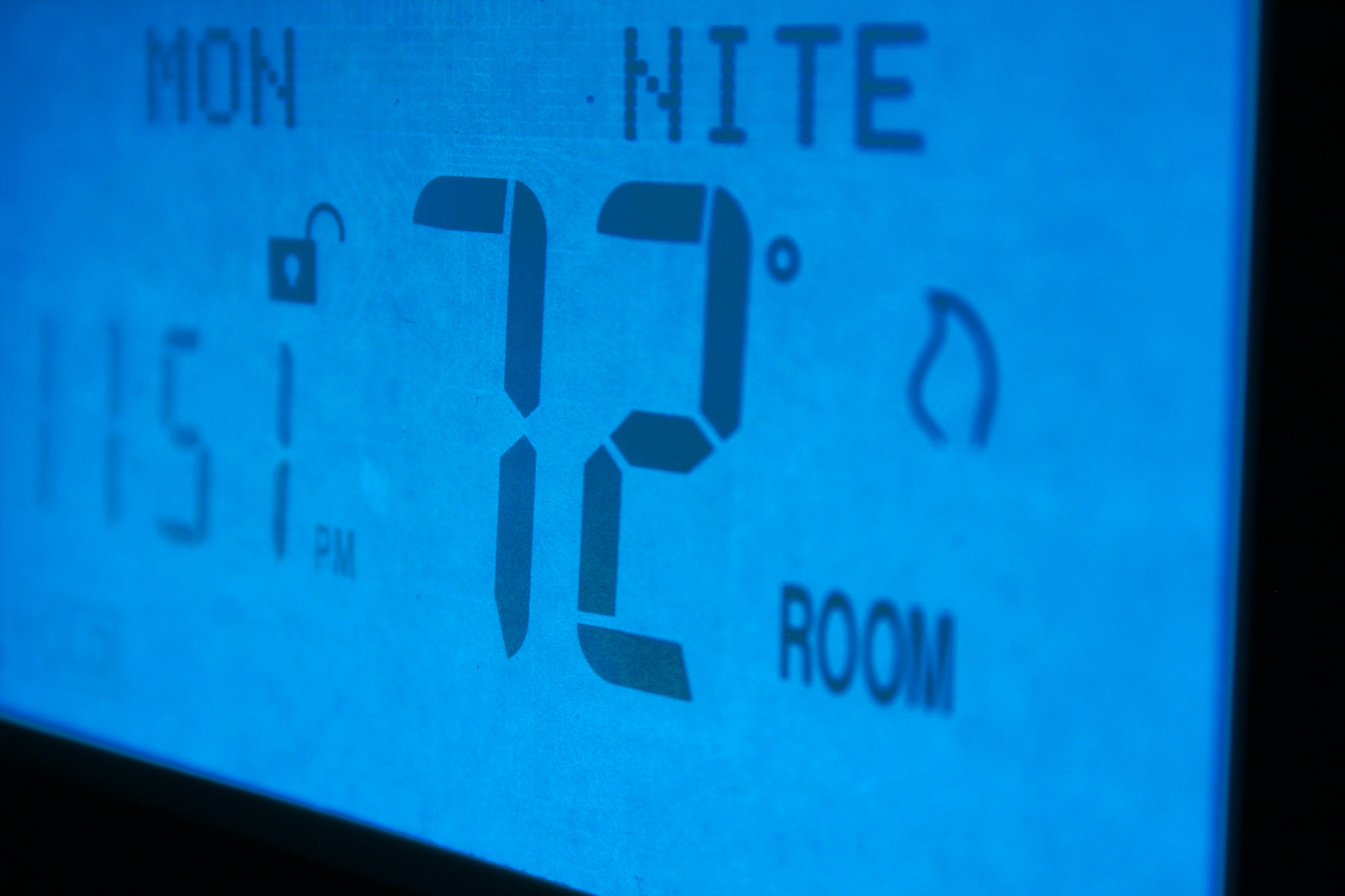This is a detailed observation of a picture of a thermostat. The thermostat is positioned at an angle, with the left side higher than the right. In the background, the bottom left corner is dominated by a black triangle, while the far right side features a vertical strip of black. The thermostat itself has a bluish-green hue. 

In the top right corner of the display, "MON" indicates that it is Monday. Directly below that, "NITE" can be seen, and one row below, it shows the time as 11:51 PM, although the "11" is notably blurry. Above the time display, there is a small icon of an unlocked lock. A much larger and more prominent display in the center shows the temperature as 72 degrees. Near the middle of the thermostat screen, there is a small flame symbol, directly above the word "ROOM."